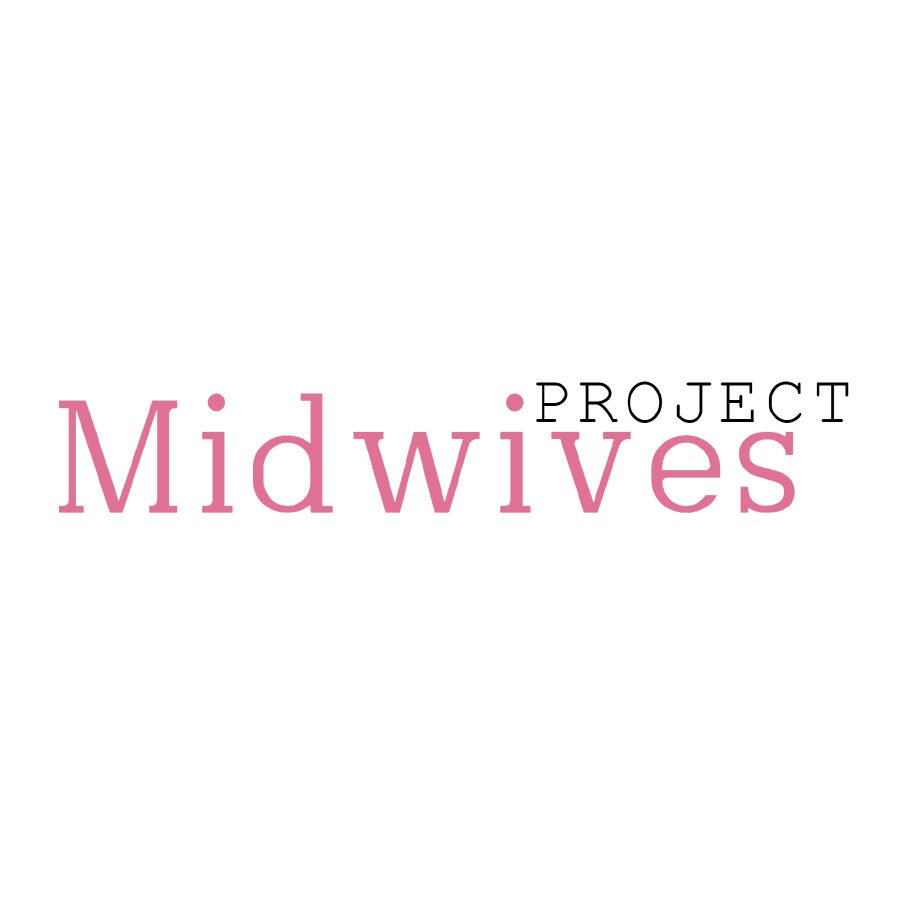The image features a white background that extends from edge to edge, with the text "Project Midwives" prominently displayed. The word "project" appears in black, typewriter-style font and is positioned towards the middle right of the image. Beneath it, the word "midwives" spans across the entire width of the image in larger, dark pink or light red letters. There are no other elements present—no photos, numbers, or additional text. This composition gives the impression of a tagline or title, possibly for a TV show or project.